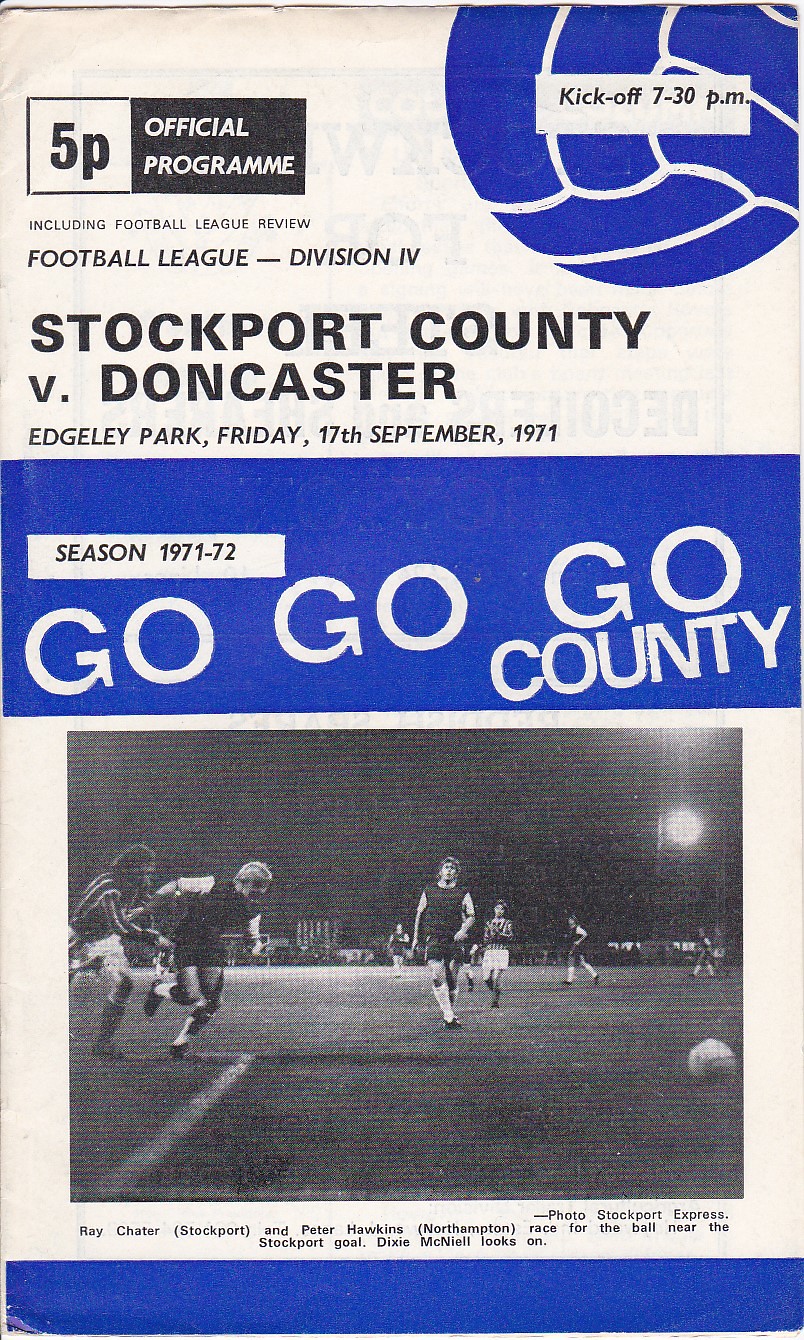This image displays the front page of a vintage soccer program or magazine, dated Friday, 17th September 1971. The primary theme is black and white, with striking blue accents. 

In the top left corner, the page is titled "5P Official Program," indicating its price. On the top right, a blue and white soccer ball is depicted along with the text "Kick off 7.30pm." 

Dominating the center is a blue horizontal banner that reads, "Go Go Go County, Season 1971-72." This promotes the featured match between Stockport County and Doncaster at Edgeley Park. 

A notable black and white photograph occupies the bottom section, showing a slightly blurred, nighttime soccer scene. The caption beneath the image reads: "Photo Stockport Express - Ray Chater Stockport and Peter Hawkins, Northampton race for the ball near the Stockport goal. Dixie McNeil looks on."